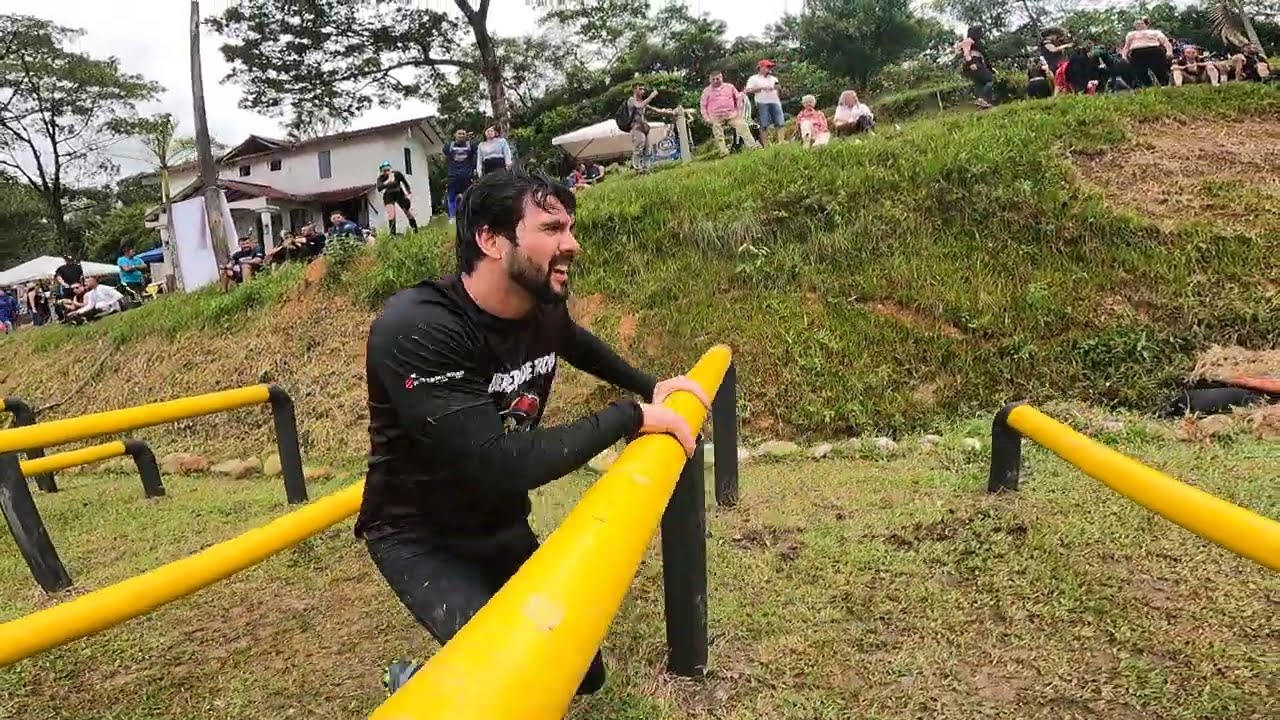This detailed photograph captures an athletic man mid-jump during an obstacle course event. He is seen running on a ground composed of green grass mixed with patches of brown soil, navigating a series of yellow and black metallic poles of varying heights. The man, who sports a black long-sleeve t-shirt adorned with white text and artwork, along with black pants, seems slightly fatigued yet focused on the challenge ahead. His beard frames a concentrated expression as he leaps over one of the yellow poles, which is supported by black posts anchored into the ground.

In the background, a grassy embankment rises behind him, occupied by a diverse group of spectators. These onlookers, estimated to be around twenty in number, range in age and attire. Some are seated while others stand, all intently watching the event unfold. Beyond this crowd, a white house can be glimpsed among scattered trees, under a sky that appears overcast and white. The overall scene is a dynamic blend of athletic effort, spectator engagement, and natural outdoor elements.